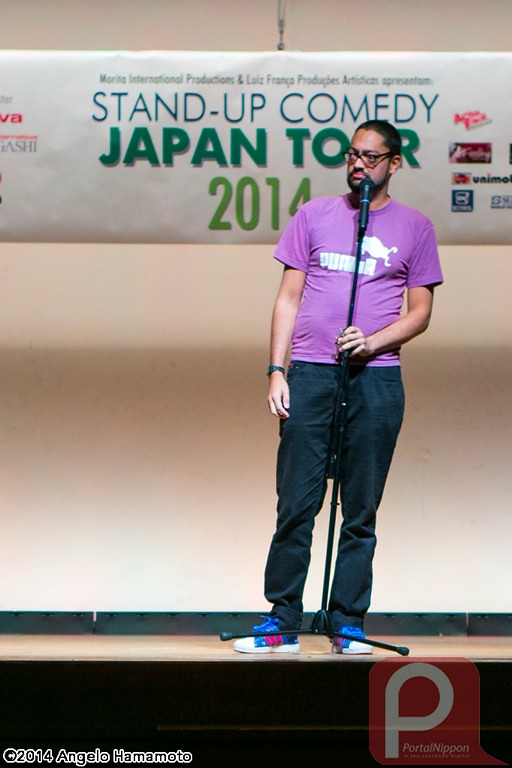In the foreground of this image, we see the front of a stage with a hardwood surface. In the bottom left corner, there's a text overlay that reads "© Angelo Amato," indicating the copyright holder. A logo is also present in the bottom right corner of the image. Centered on the stage, a man is standing at a microphone, presumably delivering a performance. 

Prominently displayed at the top left of the image, there is a poster that reads "Stand-Up Comedy Japan Tour 2014." This gives context to the scene, suggesting it's part of a comedy tour. The poster and the stage are surrounded by a variety of colors, including black, white, red, yellow, dark blue, purple, green, and teal, adding vibrance to the setting. 

The entire scene takes place indoors, but the time of day is indeterminate from the available visual cues. Overall, the image captures an engaging moment from what appears to be an ongoing comedy show.